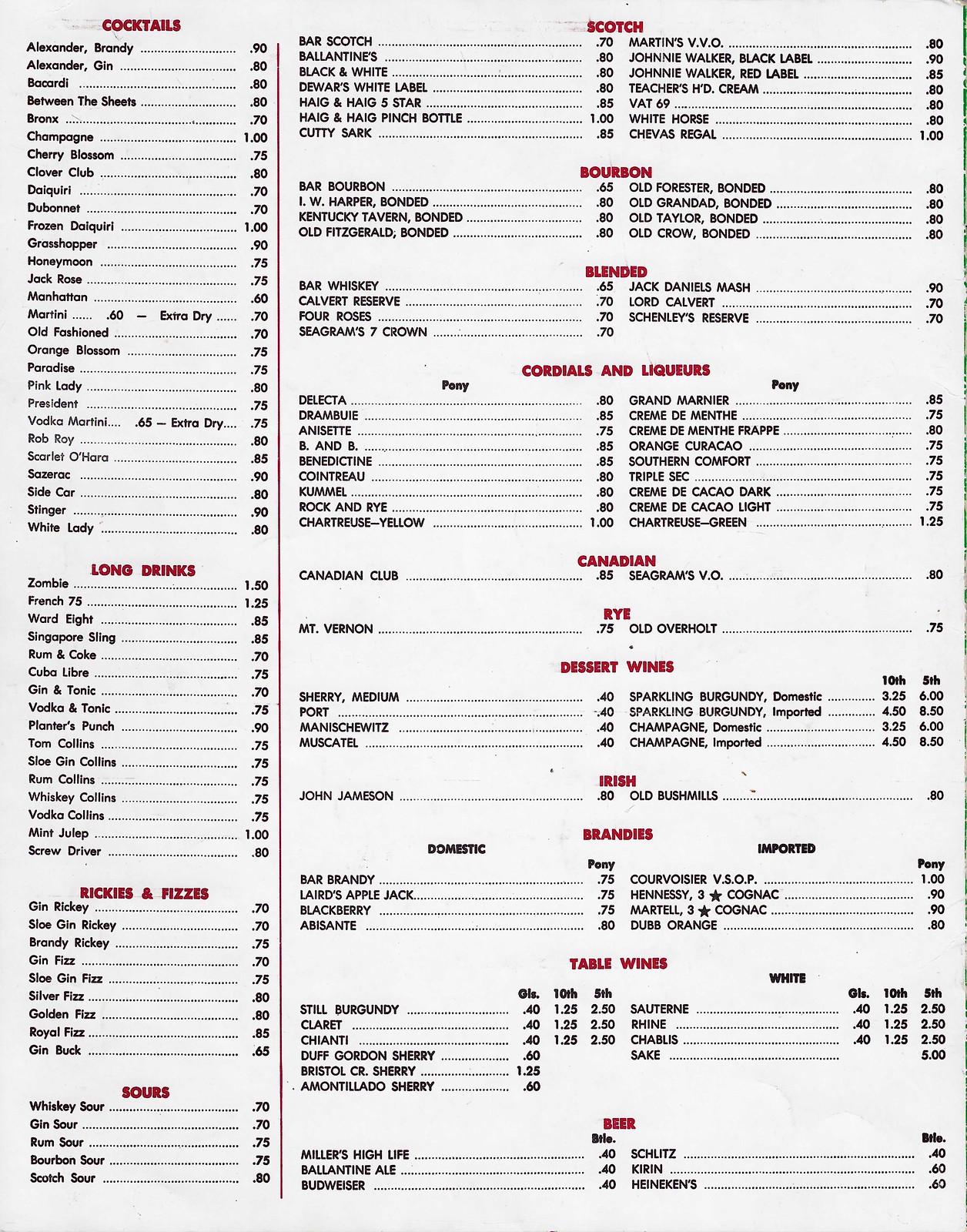The image showcases a slightly taller-than-wide menu with an off-white background. The layout is organized into two main columns separated by a distinct vertical red line. The headers, written in a dark red hue matching the vertical divider, categorize the offerings.

On the left column, starting from the upper left:
- **Cocktails**: Approximately 20 items listed
- **Long Drinks**: Around 15 options
- **Rickys and Pizzas**: About 10 selections
- **Sours**: 5 items

The right column, which is about two-thirds of the overall width, features:
- **Scotch**: This section is split into two columns, each containing 8 options.
- **Bourbon**: Consists of 4 items per column.
- **Blended**: 4 options on the left side, and 3 on the right.
- **Cocktails**: Roughly 10 items per column.
- **Canadian**: 1 option per column.
- **Rye**: 1 option per column.
- **Dessert Wines**: 4 items per column, totaling 8.

The layout and categorization bring clarity and easy navigation to the menu, ensuring an organized presentation of the beverage selections.